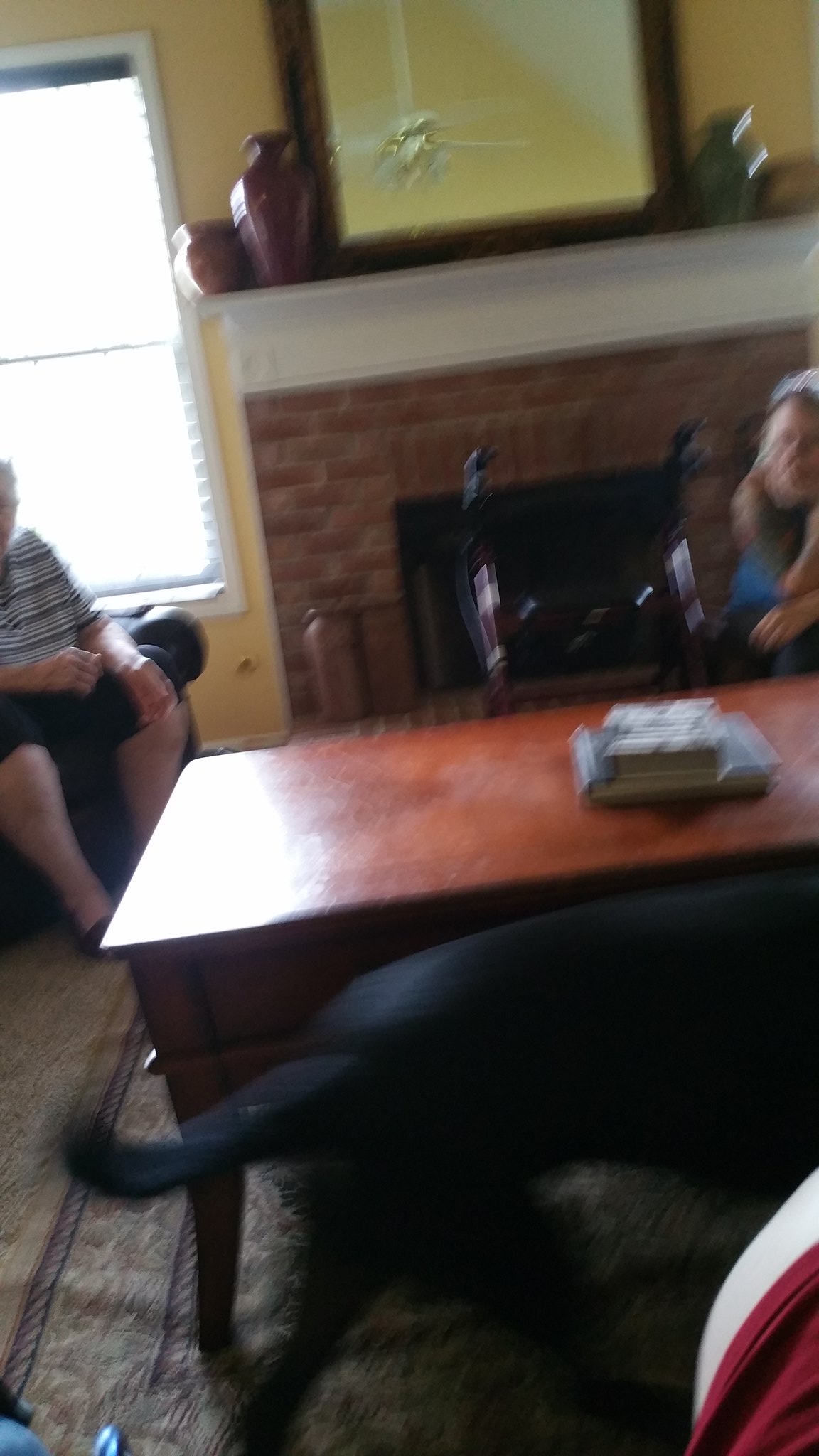A cozy living room scene features a brown wooden table adorned with an open book. In front of the table, a black dog sits attentively. The floor is covered with a plush brown carpet. To the side of the table, a person's leg, covered in a red cloth, is visible. Nearby, another person's two legs clad in black cloth and slippers are seen. Their arms, dressed in a gray and white striped shirt, rest on their lap. Above the gray-haired head of this person, which shows a surprised expression, is a black fireplace serving as the room's centerpiece. The fireplace is flanked by a large mirror above it. On the mantel, a red urn and a green urn, each likely containing cremated remains, are positioned. To the left of the scene, a window lets in natural light, adding to the room's ambiance.